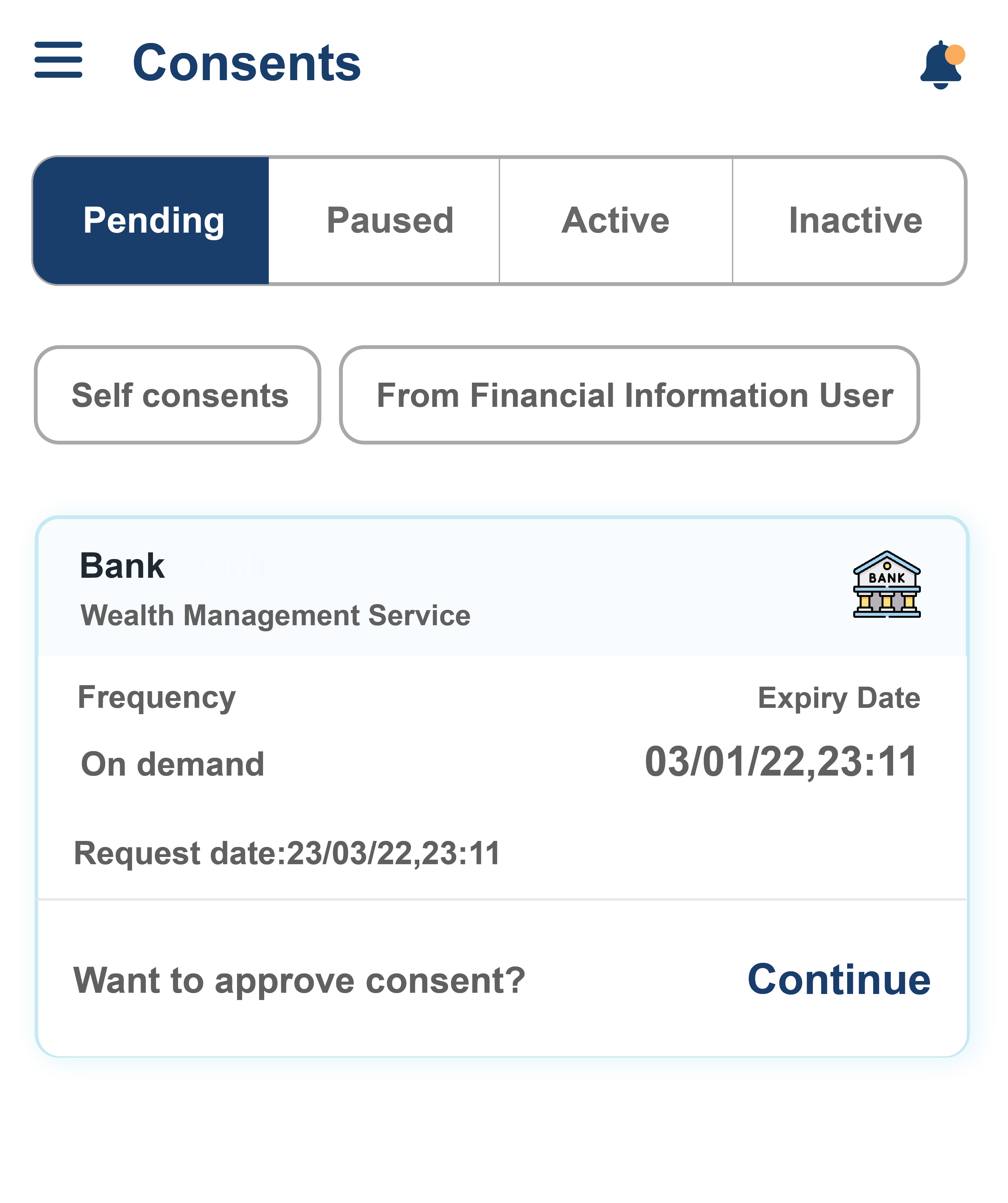A cropped screenshot of a website's consent tab is shown. At the top left, the header reads "Consents" in bold blue font. To the left of this header is a menu tab, while to the right there is an alert icon featuring a yellow circle in its top right corner. Below the header, there are four categories listed: "Pending," "Paused," "Active," and "Inactive," with "Pending" highlighted in blue.

Directly below these categories are two sections. The first section is a small bar labeled "Self-Consents" on the left, with "From Financial Information User" to its right. The second section features a blue-outlined box.

Within this box, at the top left, the text "BANK" appears in bold letters. Below this, in gray letters, it says "Wealth Management Service." At the top right of the box, there is an icon of a bank. The section continues with the label "Frequency" on the left, followed by "On Demand." To the right, it displays "Expiry Date" with a specified date and time.

At the bottom left of the box, "Request Date" is listed, followed by a specific date. Below this, there is an option labeled "Approve Consent" in gray font, and to the right, a dark blue button labeled "Continue."